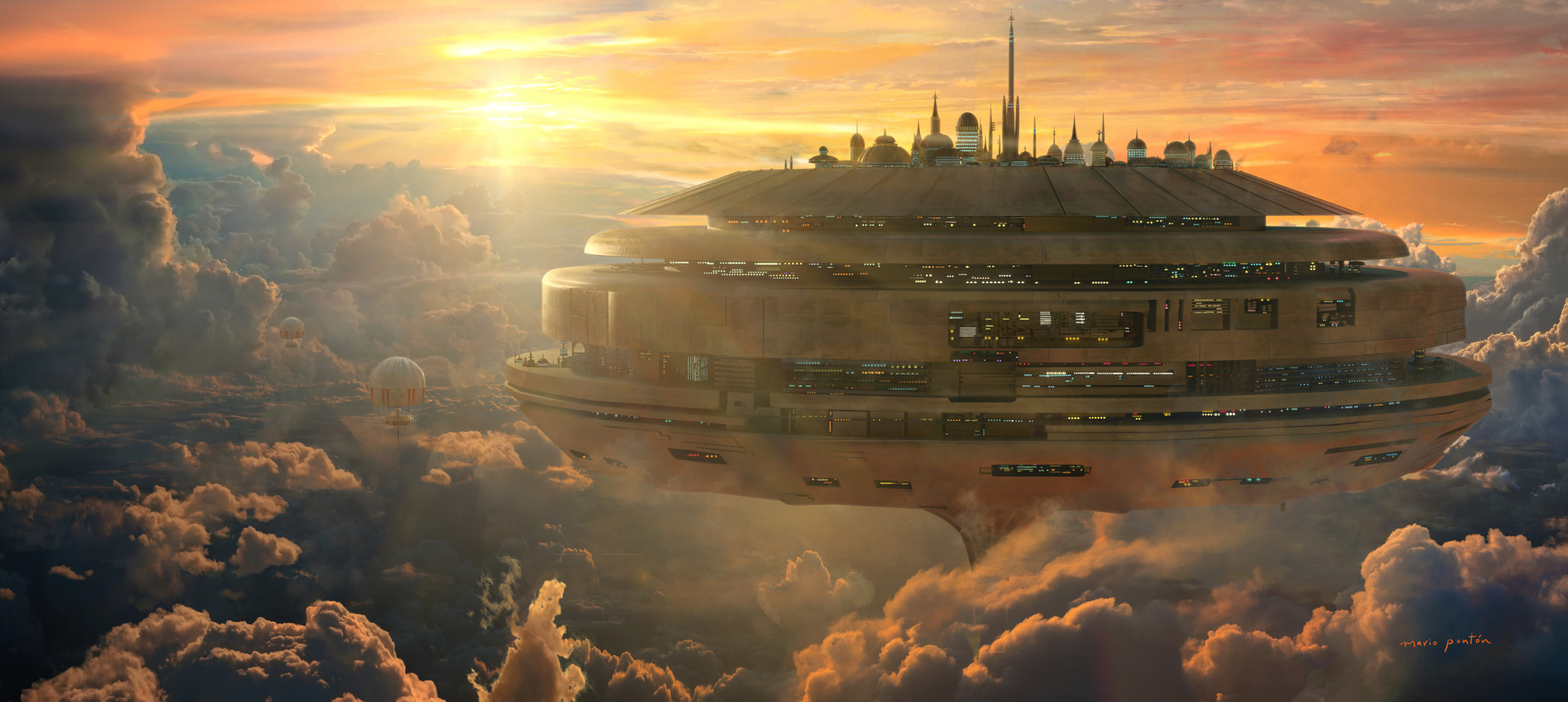The image depicts a vast, futuristic cityscape hovering above an expanse of dense clouds, reminiscent of a sci-fi setting like "Star Wars." The city is structured vertically with multiple levels, and features numerous buildings and antennae at the topmost layer. Its towering structure, somewhat similar in appearance to the Space Needle in Seattle, suggests a long base that extends down to the ground, though obscured by clouds. The city is bathed in the warm hues of a setting sun against an orange sky, which accentuates its grandeur. Floating nearby, there are at least two machines resembling hot air balloons, hinting at a high-tech mode of transport for residents. The large, circular central dome is adorned with lights and windows, indicating it might serve as a residential area or a data-collecting hub. Overall, the image portrays an enormous, bustling, and self-sustaining floating city, a beacon of advanced human civilization in a sky-high setting.